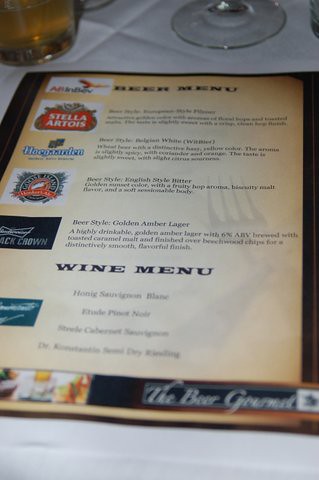This photograph captures an elegant restaurant setting, featuring a meticulously arranged table adorned with a white linen tablecloth. Visible in the frame is the base of a clear wine glass, indicative of fine dining. Adjacent to it stands a beer glass filled with an amber-colored brew, offering a hint at the variety of drinks available.

At the heart of the image lies the restaurant's menu, framed in a sophisticated brown border that encases what looks to be parchment-like paper. This particular menu highlights the beer and wine selections. Down the left-hand side, there are several beer advertisements, though not all are fully legible. They appear to include brands such as All in Bev, Della Arto, and Hargarten, with one clearly named Black Crown.

Among the featured beer descriptions, one can discern an “English style bitter” described as having a "golden sunset color with a fruity hop." The other detailed listing is for a “golden amber lager” boasting a "highly drinkable golden amber lager with 6% ABV, brewed with toasted caramel malt, and finished over beechwood chips for a distinctively smooth, flavorful finish."

Additionally, the wine menu is present, although details are not specified in the image. This carefully crafted menu and its surrounding elements underscore the upscale ambiance of the dining experience.